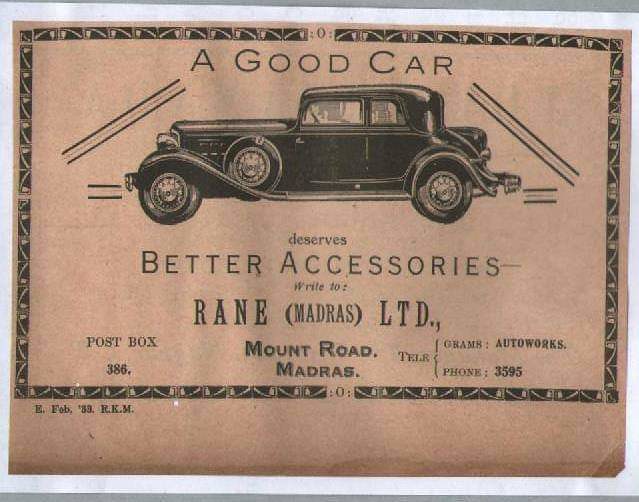In this vintage black-and-white advertisement, a prominently framed old car is depicted in a classic side view, with the front of the car facing left. The paper, which appears aged with a yellowish tint, features multiple borders—an inner black border covering the top seven-eighths of the sheet, followed by white and gray framing. Above the car, the text “A good car” is styled in a black banner. Below the vehicle, the text continues with “deserves better accessories” followed by the company details: "Rain Limited, Post Box 386, Mount Road, Madras." Additionally, the ad features other inscriptions such as "grams: autowork, phone: 3595." The overall design suggests it is from the 1940s or 1950s, emphasizing the quality of car accessories offered by Rain Limited.